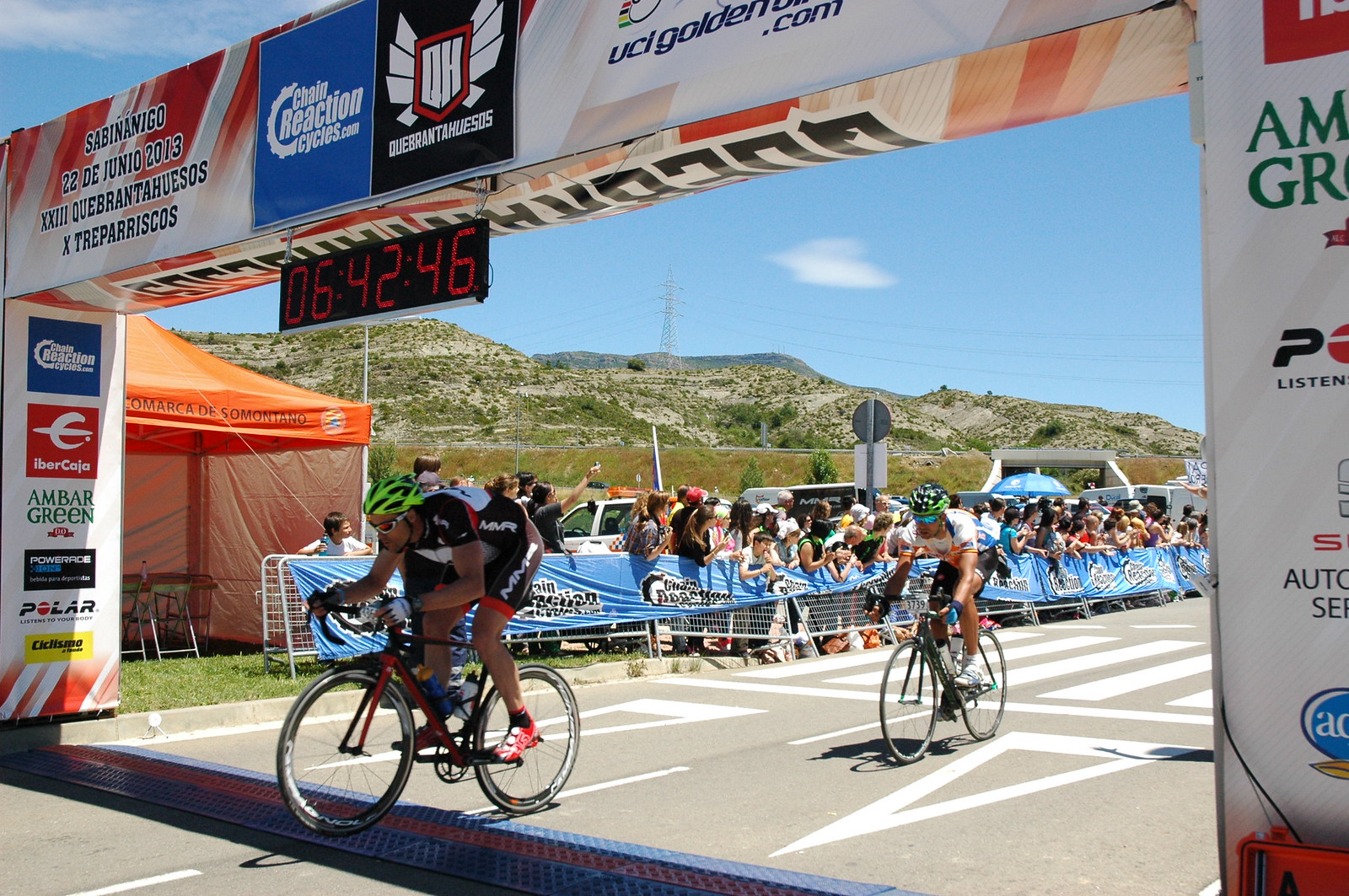The photograph captures the concluding moment of a competitive bike race as two cyclists cross the finish line. The finish line is marked by a large archway or scaffolding adorned with a white background and colorful sponsor logos, including Powerade, Polar, Ambar, and ChainReactionCycles.com. The archway prominently displays a digital clock showing the race time of 6 hours, 42 minutes, and 46 seconds. Below the archway, the road, which is gray with white lettering, leads the racers to their final sprint. One cyclist, dressed in an entirely black outfit, and another wearing a white shirt with black shorts, both sporting green helmets, push towards victory. Spectators line the sides of the road, standing behind bright blue barriers, collectively cheering on the finishers. The backdrop features scenic mountains and a partly cloudy sky, adding to the triumphant atmosphere of the event held on June 22, 2013.